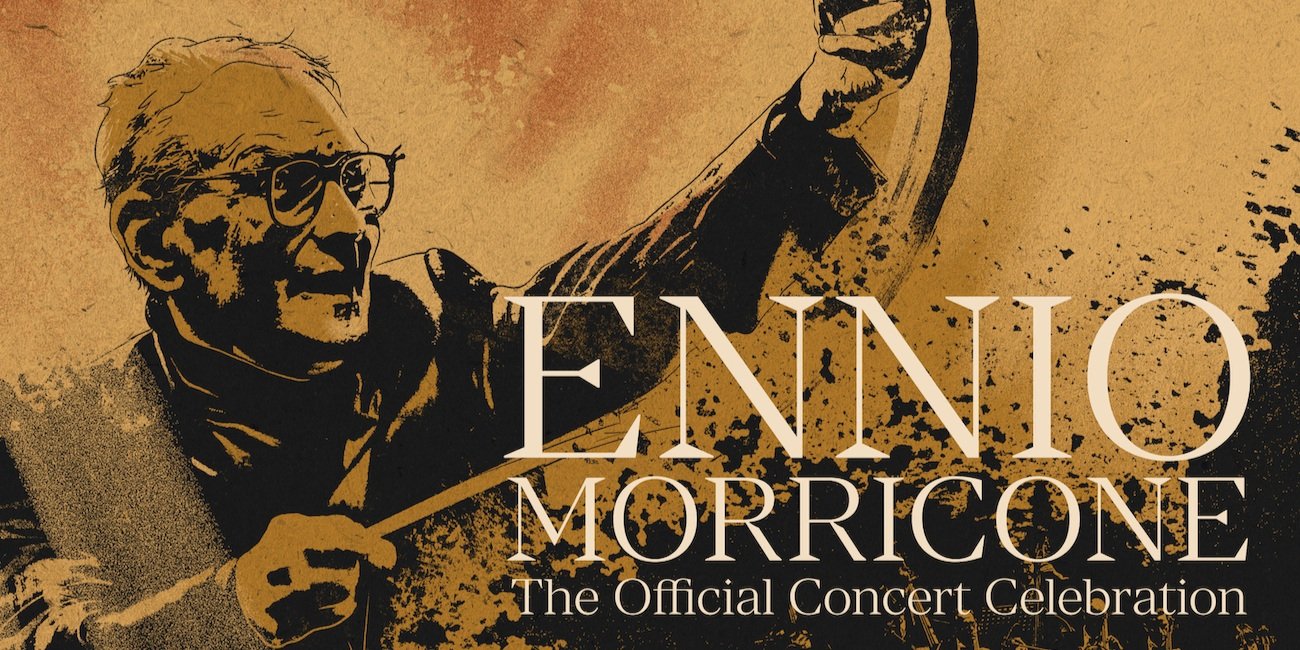This rectangular landscape-oriented image appears as a rustic, print-style painting, approximately 5 inches wide and 3 inches high. The background varies in shades of light brown, beige, and dark tan, with touches of reddish-brown particularly in the lower right-hand corner. Black splashes and speckles are scattered across the background, giving it a loosely painted, textured appearance.

Dominating the left side of the image is the black-outlined figure of an elderly man, depicted from the chest up. He is facing towards the right side, wearing large glasses, a turtleneck, and a jacket. His balding head features light hair, and his left arm is raised, extending out of the picture's top edge, while his right arm is bent at the elbow, holding a conductor's baton.

The focal point is accentuated by the text in large white letters in the lower right-hand corner, spelling out "Ennio Morricone" with “The Official Concert Celebration” beneath it in smaller white print. The image effectively combines the detailed depiction of the man, presumably conducting, with a dynamically textured and colored background, evoking a sense of both formality and artistic fluidity.